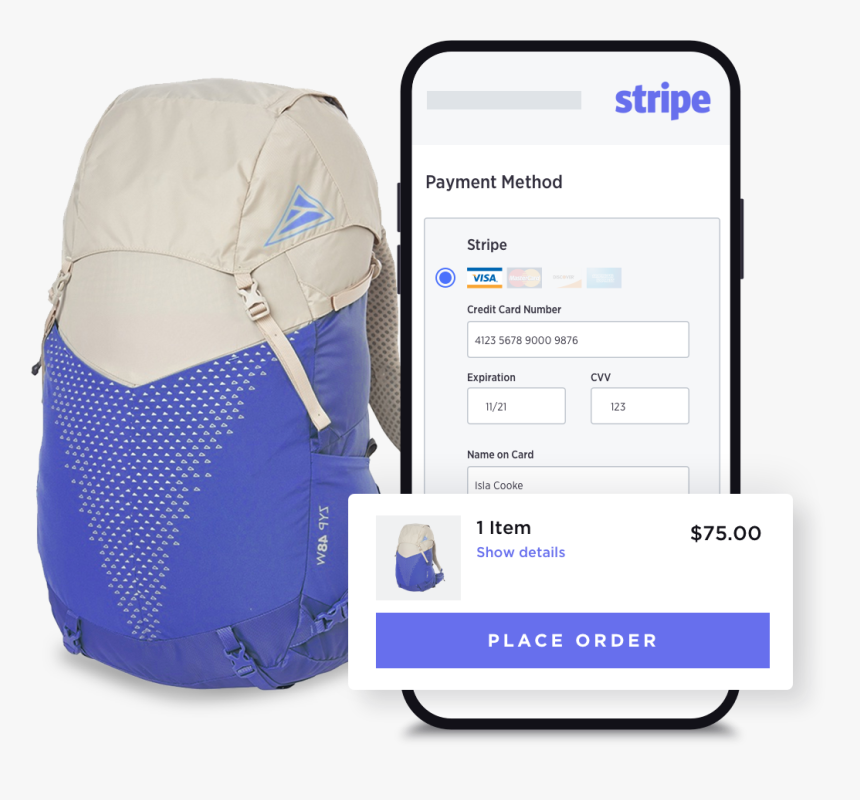The image depicts a user interface from an online store set against a white background. On the right side of the interface, the top right corner features the word "STRIPE" written in purple. Below this, there is a text section labeled "Payment Method," also set against a white background, with "STRIPE" as the detailed option below it. The selected payment method is a VISA card, displayed in blue, white, and yellow. Additional payment options, including MasterCard and two other transparent methods, are shown on the right. MasterCard is written in white with an orange and yellow logo.

Further details of the chosen VISA card include the credit card number 4123 5678 9000 9876, an expiration date of 11/21, a CVV of 123, and the name on the card, Isla Coke. At the bottom of the interface, there's a pop-up indicating an item priced at $75. The phrase "Show Details" is written in purple, and the item description reveals it to be a bag. 

The bag is displayed on the left side of the image; it has a cream white top and a blue bottom with cream white triangle dots in the center. The bag is oriented towards the left. Below the item pop-up, there is a purple button labeled "Place Order" in white text. To the side of the bag, the code "ZYP48W" is printed in white.